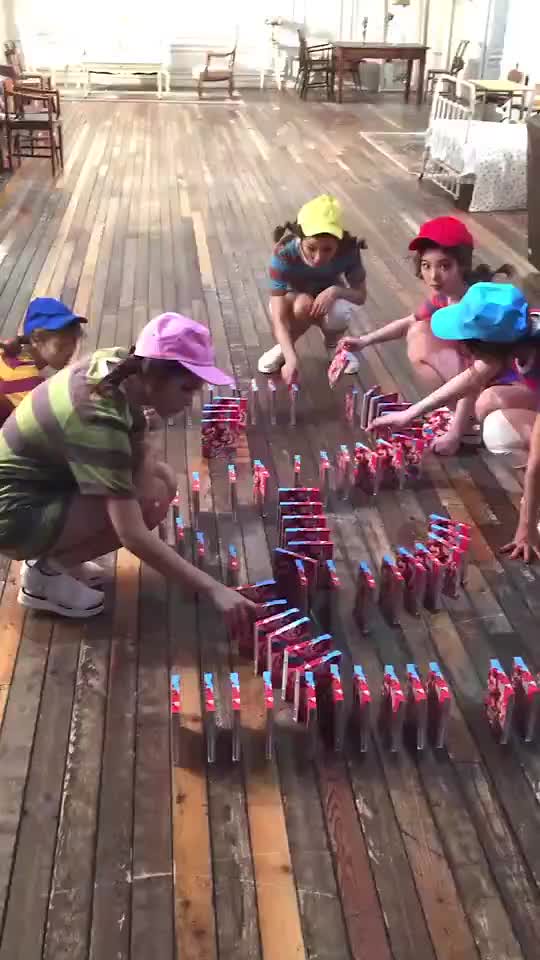This is a colour photograph in a very stretched portrait orientation, capturing several children deeply engrossed in a collective activity. The children are all crouched down with their knees fully bent so that the backs of their thighs rest on their calves, and their chests are nearly touching their knees. They are positioned on a large wooden surface that runs from the top to the bottom of the photo, consisting of mismatched wood panels in dark browns, reddish browns, and light pine shades, which appears to be a deck or porch.

The children are arranging large, red and blue rectangular objects, somewhat the size of CD cases, in intricate, snaking lines reminiscent of a domino setup. Although the objects don't resemble traditional dominoes or toy soldiers, they are clearly intended to create a cascading effect when one is knocked over, setting off a chain reaction.

Each child wears a baseball cap of a different colour—pink, dark blue, turquoise, yellow, and red—and a variety of T-shirts. Specific outfits include a grey and green striped T-shirt, a yellow and maroon striped T-shirt, and a blue and maroon striped T-shirt. One child also seems to glance towards the camera. The background is heavily overexposed, making it difficult to discern whether they are indoors or outdoors, but it seems like there could be furniture like chairs and tables in the far distance.